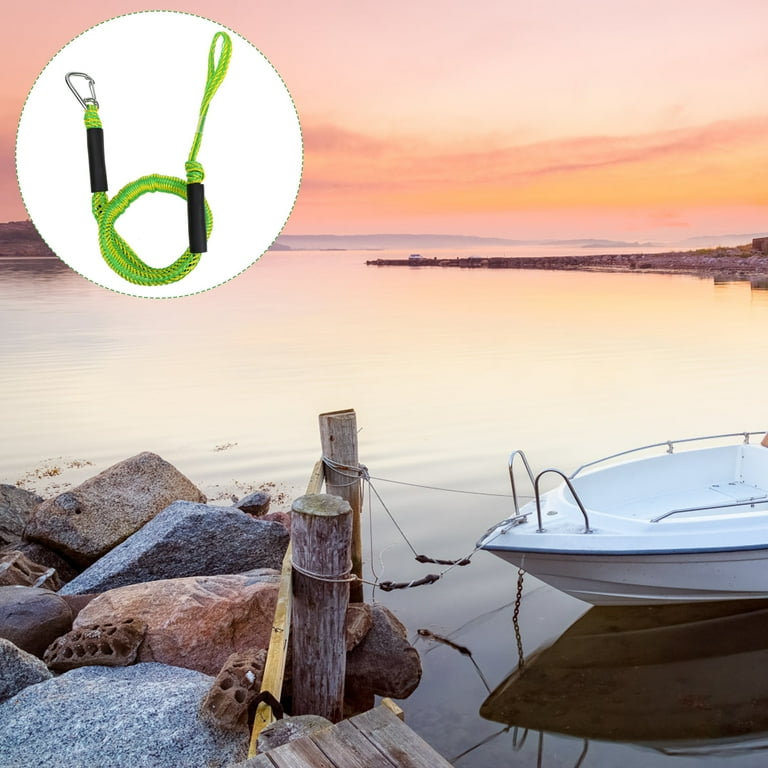This image captures a tranquil scene of a calm lake or ocean, with the water mirroring a stunning purple, pink, and orange sunset sky. The water, appearing almost white with subtle glimmers of these vibrant hues, is incredibly flat and clear, with gentle ripples. In the foreground, there's a wooden dock with a wooden pole tied to which is the front half of a small white boat, likely a two-seater intended for fishing. The serene water flawlessly reflects the boat. Additionally, at the top-left corner of the image, there is an overlay featuring a product—a green rope with a silver carabiner, suggesting it might be the same rope used to secure the boat, demonstrated within a dotted green circle on a white background, adding an informative dimension to the picturesque view. Scattered boulders also adorn the nearer surroundings, enhancing the natural and peaceful ambiance of the scene.